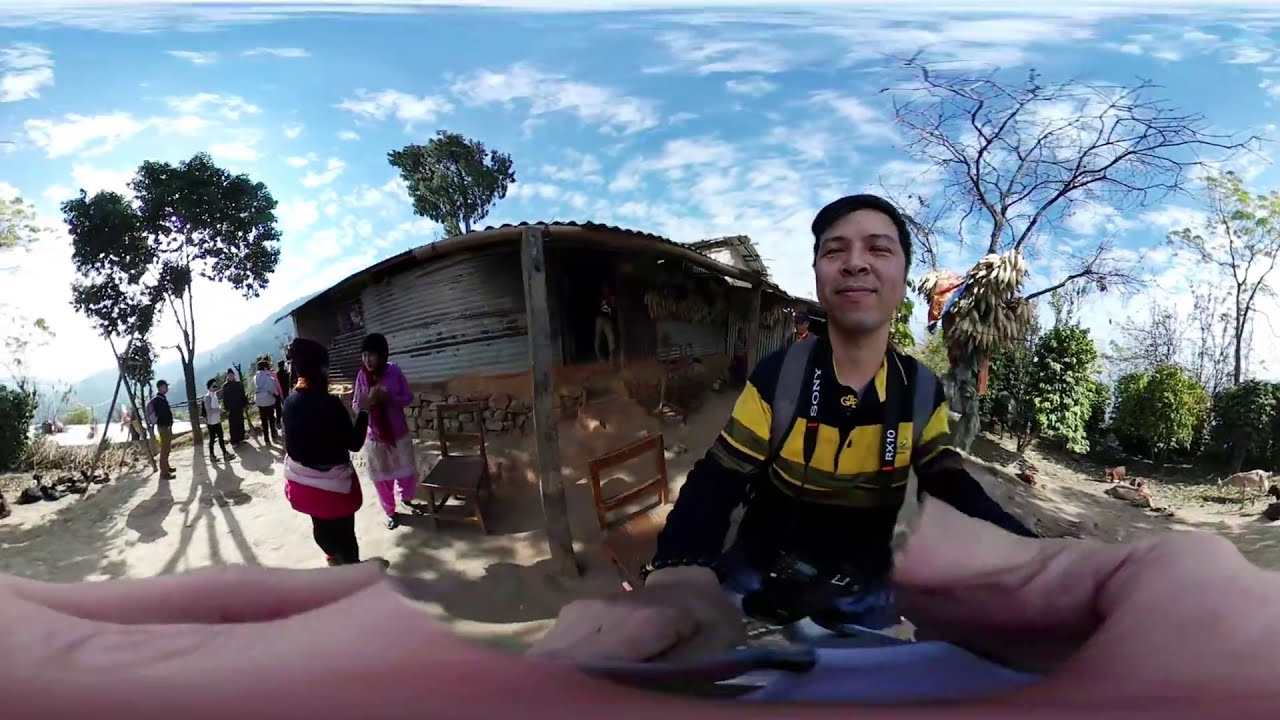The distorted, fish-eye image captures an outdoor setting, likely a village or a historical site, under a blue sky dotted with white clouds. At the center-right, a man with short dark hair and a cheerful expression stares into the camera, wearing a black shirt with yellow stripes, and a Sony lanyard around his neck. He appears to be the photographer, his hand positioned at the bottom of the image and a backpack visible by the straps around his shoulders. To his left, two women are engaged in conversation against a backdrop that includes several groups of people, some carrying backpacks. The ground beneath them is sandy or dirt-colored. Prominently in the middle, there's a curved, old tin building with a metal roof supported by wooden beams, adding to the rustic atmosphere. Alongside, there are old wooden chairs and in the surrounding area, different kinds of trees, including a bare tree to the right and banana trees on the left with large bunches of bananas hanging.